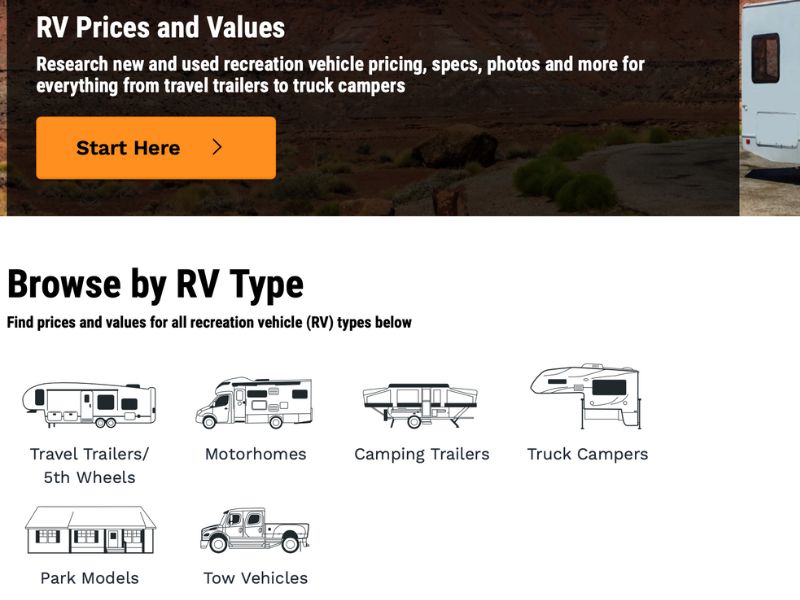The image captures a detailed section of an RV pricing website. At the top, a banner spans across the screen, featuring a vibrant rocky canyon as its background. Emerging from the right side of this scenic backdrop is an RV, partially cropped due to the close-up nature of the image. The banner overlays white text that reads, "RV Prices and Values," followed by a subheading that elaborates, "Research New and Used Recreation Vehicles, Pricing, Specs, Photos, and more—for everything from travel trailers to truck campers."

Below this informative banner, an eye-catching "Start Here" button in bright orange is prominently displayed, featuring black font. The main section of the webpage, set against a white background, is titled "Browse by RV Type," positioned on the left. Under this heading, a list of six RV types is presented in a sequential order, with the first being "Travel Trailers." The organized layout and detailed descriptions guide users in navigating their RV research and decision-making process.